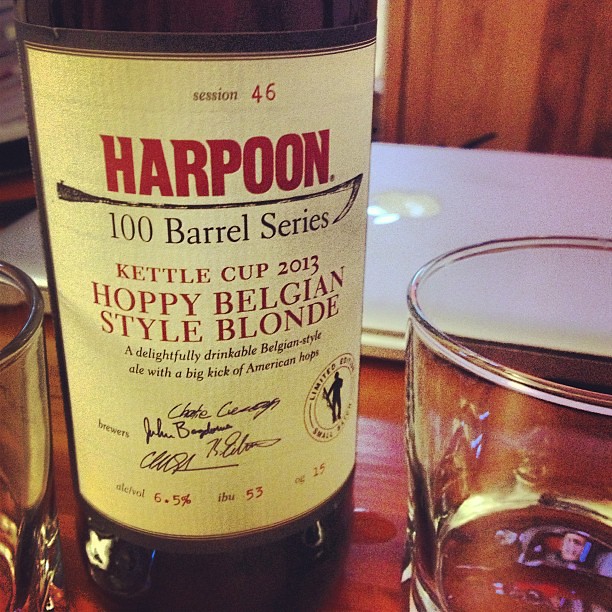This image showcases a detailed close-up of a Harpoon 100 Barrel Series Kettle Cup 2013 Hoppy Belgian Style Blonde beer bottle, prominently placed on a light wooden table with a matching light wooden wall backdrop. The bottle, which is primarily black, features a tan label adorned with red and black text. At the top of the label in red, the text reads "Session 46," followed by the name "Harpoon" underlined by a drawing of a harpoon. Below, in black print, it states "100 Barrel Series," and further down it says "Kettle Cup 2013, Hoppy Belgian Style Blonde." Additional text describes it as "a delightfully drinkable Belgian style ale with a big kick of American hops." Signatures of the brewers are visible beneath this text. To the left of the bottle, an outline of an empty glass can be seen, while to the right, there is another empty glass sitting close by. Both glasses appear to have a silver hue and are positioned on the same wooden table which occupies the bottom two-thirds of the image. Additionally, a MacBook laptop with its lid shut is placed in the background, subtly visible on the table. The overall scene captures a refined setting showcasing the distinctive bottle and its detailing.